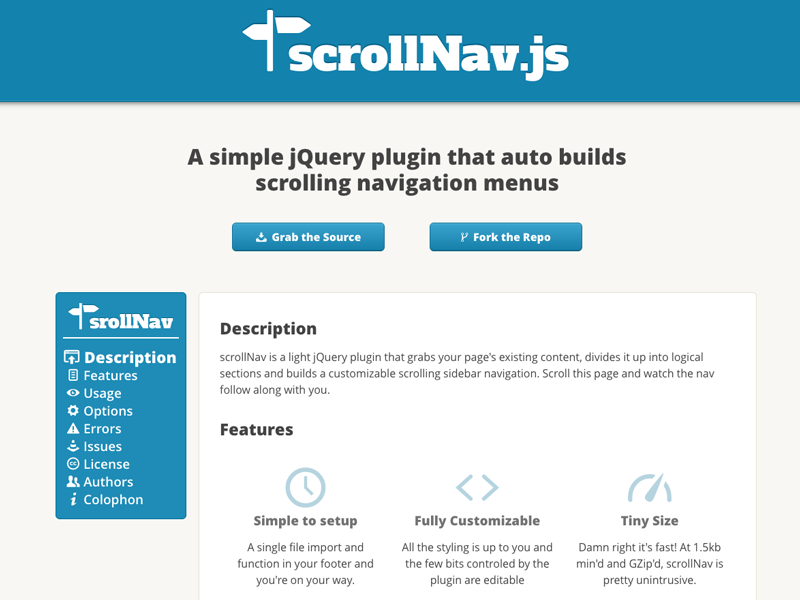Screenshot of ScrollKnob.js Website

The screenshot captures the homepage of the ScrollKnob.js website, which features a clean, white background. At the top, there is a blue banner prominently displaying the website's logo in white, which resembles a poll with two signs and the name "ScrollKnob" also in white.

Below the banner, a succinct caption describes ScrollKnob.js as "a simple jQuery plugin that auto-builds scrolling navigation menus," effectively summarizing the site's purpose. Just underneath this caption, two blue buttons are positioned side by side. The button on the left, labeled "Grab the Source," includes an icon, while the one on the right, labeled "Fork the Repo," also comes with its own icon.

In the bottom left corner of the page, there is a tool column titled simply "ScrollKnob" (notably missing the "C" from the full website name) and accompanied by the website's icon logo. This column features a white dash followed by an organized list of icons and headings, each representing different sections of the website: Description, Features, Usage, Options, Errors, Issues, License, Authors, and Colophon.

To the right of the tool column, a bolded description reiterates the plugin's functionality. It emphasizes that ScrollKnob is a lightweight jQuery plugin designed to automatically categorize existing page content into logical sections. The description is followed by a bolded "Features" section, which showcases three key attributes of the plugin using distinctive symbols: it is simple to set up, fully customizable, and has a tiny size. Brief descriptions accompany each feature, succinctly explaining the plugin's user-friendly setup, customization options, and minimal footprint.